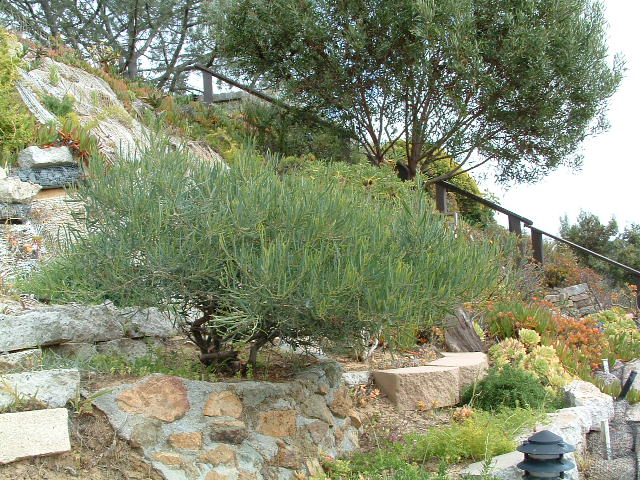The image depicts a lush and verdant hillside, carefully terraced with both beige and gray stone platforms studded with various plants and flowers. Dominating the center of the photograph is a large green bush with stringy leaves and dark brown branches, set on a slope. The slope is also punctuated by a small, unlit lamp positioned near the bottom of the image, which would illuminate the footpath at night.

In the background, a black or brown stair banister ascends the hillside, suggesting the presence of a staircase, although the steps themselves are not visible. This banister likely leads to an area with a building. The entire scene takes place in a broadly wooded area, enriched with several trees, including one prominent tree at the center and another in the background. 

The sky is bright and white, with hints of blue indicating a sunny day. The photograph showcases a beautiful and green outdoor setting, highlighting the natural beauty and careful landscaping of what appears to be a garden or park area.